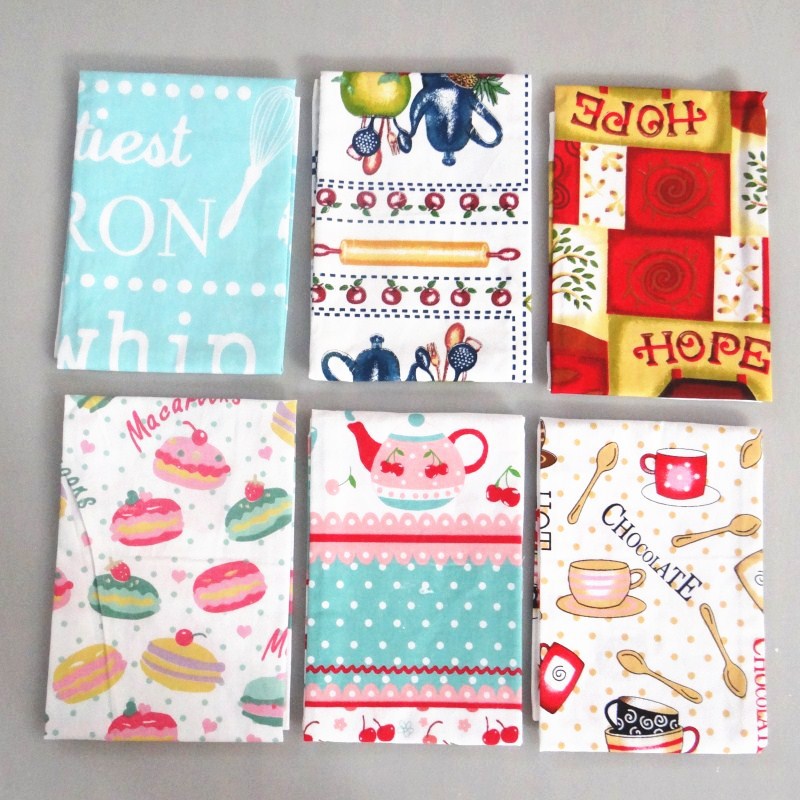This detailed photograph features six neatly folded dish towels or tablecloths, arranged in two rows of three, resting on a grayish kitchen countertop. Each towel showcases unique and colorful designs with kitchen themes:

1. The top left towel is a light blue fabric adorned with white writing and illustrations. The word "whip" and an image of a whisk are visible amidst scattered white dots.
2. Next to it, the second towel has a whimsical country motif on a white background, including a rolling pin, little apples, a teapot, and an apple-shaped utensil holder filled with assorted kitchen utensils.
3. The top right towel is predominantly red with a gold border and white sections, displaying the word "hope" in red text at both the top and bottom.
4. The bottom left towel features various colorful macarons on a white background with purple dots.
5. To its right, the fifth towel has a design of a teapot on a predominantly white background, intermixed with pink, red, and teal accents and white dots.
6. The bottom right towel showcases a white fabric with yellow dots, decorated with images of spoons, coffee mugs, and the word "chocolate" inscribed in black.

Each towel is meticulously folded, highlighting their distinct kitchen-themed prints and bringing a playful touch to the countertop backdrop.